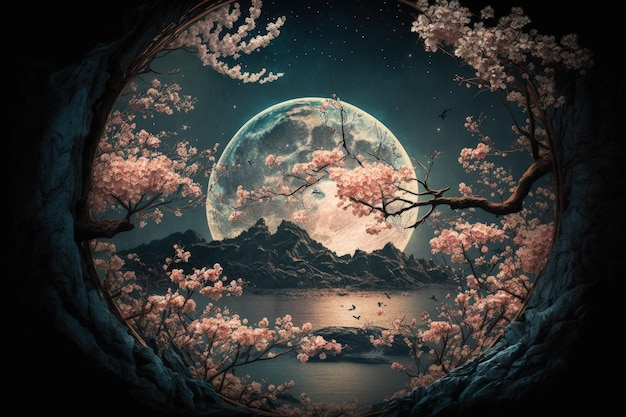This image is a highly realistic artwork, either hand-painted or computer-generated, capturing a serene nighttime scene. The composition reveals a view from within a cave-like structure, framed by rocky outcrops on both sides. Emerging from this circular aperture, the foreground is adorned with trees in full bloom, their branches heavy with vibrant pink and white cherry blossoms cascading around the edges. Central to the scene is a bright, full moon that hovers just above a rugged mountain range, casting a luminous glow over the tranquil landscape. In front of the mountains lies a shimmering lake, which mirrors the moonlight. The waters are dotted with birds, and one bird is visible flying close to the moon. The night sky, painted in deep blues and blacks, is speckled with twinkling stars, enhancing the ethereal quality of the setting. The meticulous detail in the flora, the lunar glow, and the serene water bodies evoke a sense of peaceful solitude and natural beauty.